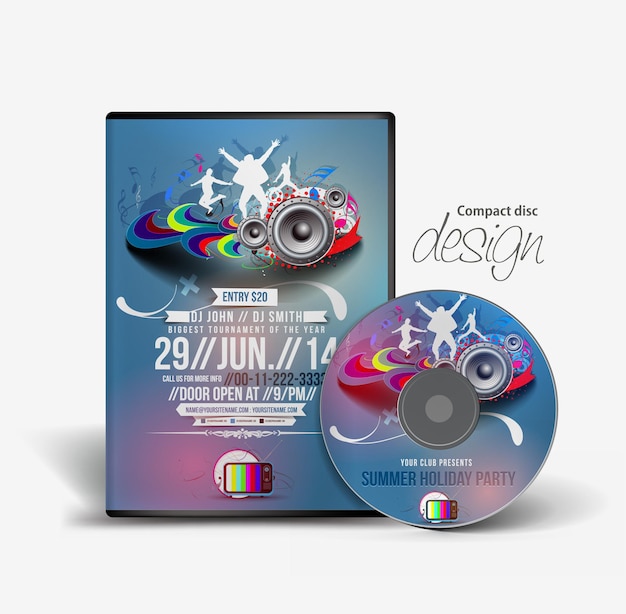This image features a mock-up showcasing a promotional design for a compact disc and its case. The primary background of the display is gray. The CD case has a striking blue cover adorned with white silhouettes of three people dancing, positioned in front of two speakers, and surrounded by an array of vibrant, curvy colored patterns in hues of yellow, blue, red, purple, and orange. The upper part of the case includes a black border and text in various styles: a blue banner with "Entry $20" in white text, followed by "DJ John" and "DJ Smith," advertising the "Biggest tournament of the year" on "29 June 14." Additional information such as a phone number "Call us for more info: 00-11-222-3333" and "Doors open at 9 p.m." are also included in white text. The bottom of the CD case and the disc display a white circle with a blue-purple outline, depicting what looks like an old TV set with color bars and control dials, serving as a logo. The CD itself, leaning against the case, mimics the cover's design with the same dancing silhouettes and speakers, and adds the text "Your Club Presents" in white, and "Summer Holiday Party" in blue. The phrase "Compact Disc Design" hovers above the CD in sans-serif and script fonts, enhancing the professional appearance of the mock-up. This design likely serves as an example of customizable CD packaging for potential clients.